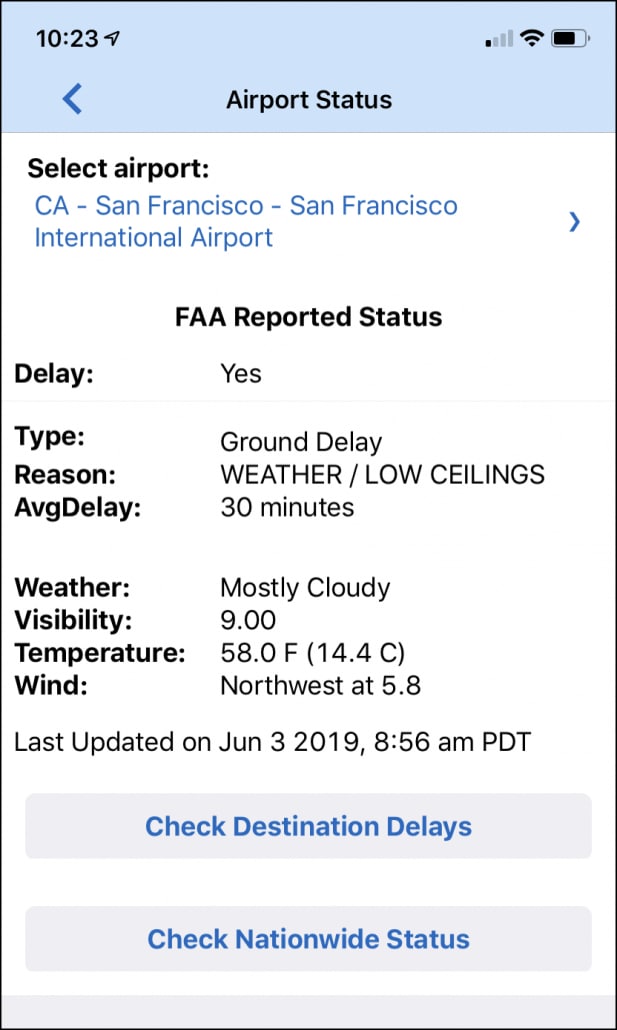Screenshot taken from an iPhone displaying airport status information at 10:23 AM. The iPhone's status bar at the top shows the location icon activated, cellular signal at 1 out of 4 bars, full Wi-Fi signal at 3 out of 3 bars, and a battery level approximating 82%. Below, the background turns predominantly white, starting with the text "Select Airport". Listed under this is "CA-San Francisco-San Francisco International Airport" with a right-facing arrow beside it.

The middle section is titled "FAA Reported Status" in bold black letters. The detailed report indicates:
- Delay: Yes
- Type: Ground Delay
- Reason: Weather / Low Ceilings
- Average Delay: 30 minutes
- Weather: Mostly Cloudy
- Visibility: 9.00 miles
- Temperature: 58.0°F (14.4°C)
- Wind: Northwest at 5.8 mph

The last update was recorded on June 3, 2019, at 8:56 AM Pacific Daylight Time.

At the bottom of the screen, there are two rectangular gray buttons with blue font options: "Check Destination Delays" and "Check Nationwide Status".